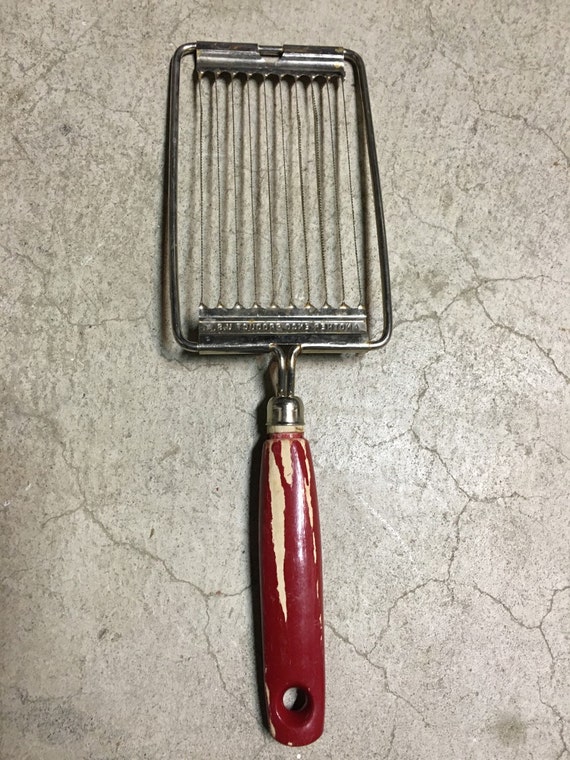This is an aerial close-up photograph of an antique kitchen tool, likely used for slicing or grating food items such as cheese, vegetables, or potatoes. Positioned on a cracked, worn concrete surface, the tool features a weathered red wooden handle with visible paint wear, revealing the natural wood underneath. The metallic section is a rectangular frame, housing ten fine vertical wires designed for cutting or grating. The frame shows signs of age with traces of rust, suggesting it has been well-used over the years. An engraved label on the metal's surface adds to its vintage charm, though it is difficult to read due to wear.